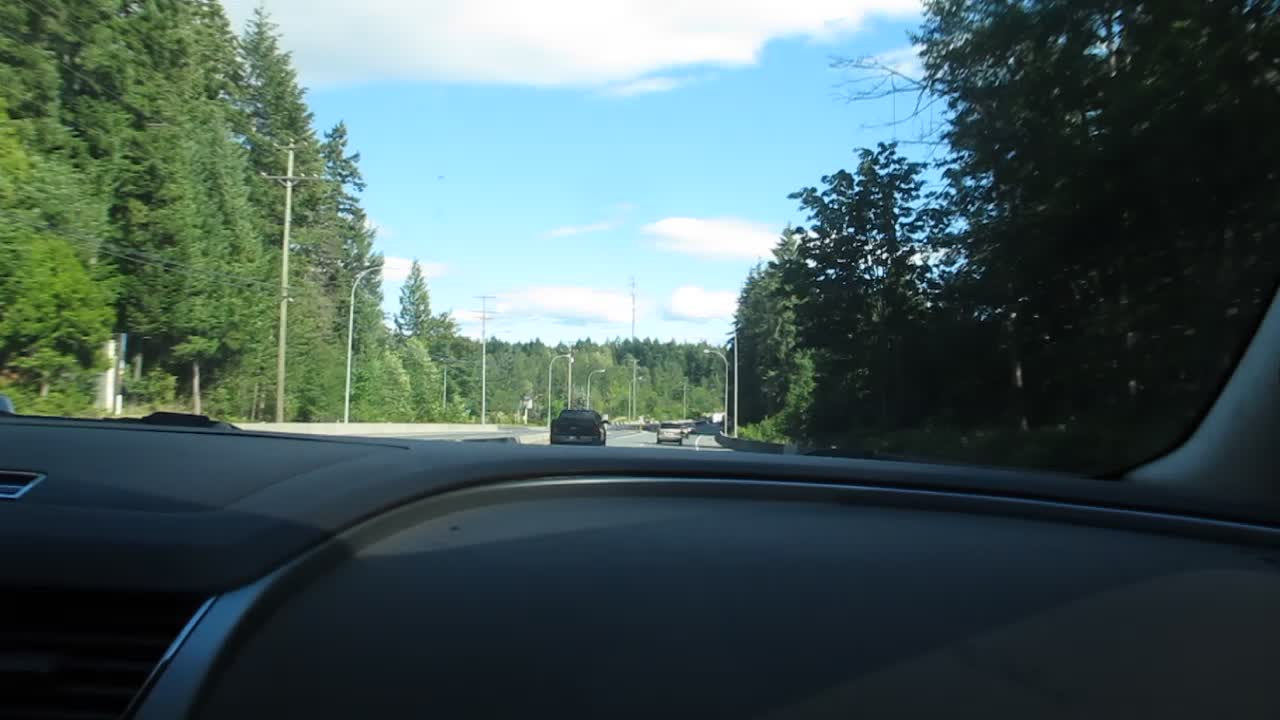A detailed photograph taken from the front passenger seat of a car driving down a two-lane highway on a partly cloudy, bright day. The interior of the car features a gray dashboard with a silver-trimmed glove compartment and a gray door frame visible on the right side, confirming the passenger perspective. The image captures a stretch of road with a few vehicles ahead, including a black truck in the left lane and a tan car farther in the distance. The highway is flanked by lush, green trees, predominantly tall evergreens, with the foliage suggesting summer or late spring. Utility poles, power poles, and light poles line both sides of the straight road. The sky transitions from a bright electric blue at the top to white near the horizon, dotted with puffy white and slightly gray clouds, indicating a possibility of rain.